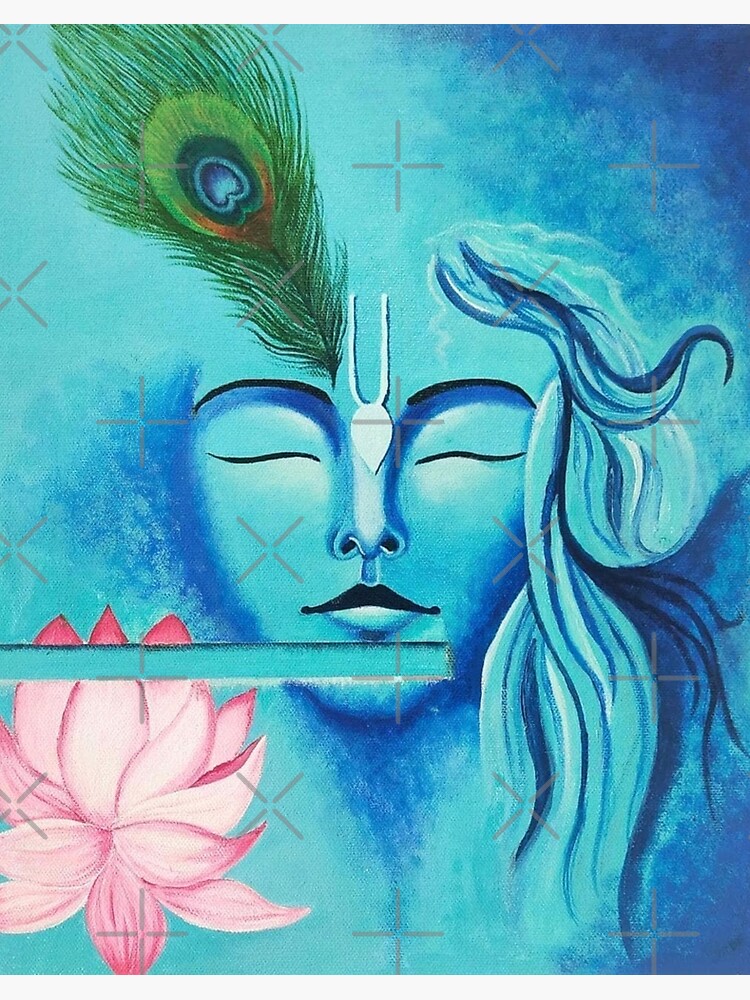This intricate and artistic drawing prominently features a woman's face centered in the composition. Her closed eyes, stylized to resemble gentle waves, add a serene expression. The nose is distinctively shaded, with a blend of white and blue tones on either side, accentuating its structure. Her lips are striking, with the upper lip rendered in black and the lower lip in blue, matching the overall blue hue of her face. Adorning her cheeks and chin are grey X marks, a motif that extends throughout the image, creating a cohesive, textured effect.

Her hair, flowing off the left side, is a mix of light and dark blue shades, enhancing the ethereal quality of the artwork. In the center of her nose, there's a white "U" shape with a teardrop-shaped white object nestled within it, adding an element of intrigue. Further enhancing the left side of the image is a green feather interwoven with hints of orange and blue, adjacent to a delicate pink flower. These elements contribute vibrant splashes of color and organic shapes to the composition, enriching the visual narrative.